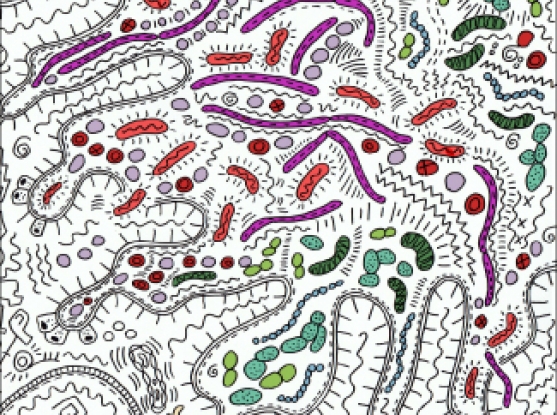The image appears to be a detailed, computer-generated illustration of a variety of microscopic life forms, potentially bacteria. Set against a stark white background, the image showcases an array of vibrantly colored organisms, including rod-shaped bacteria, elongated forms, circular structures, and snake-like figures. The bacteria vary in color, with hues of red, green, dark green, light green, purple, blue, and black. Some of the red bacteria resemble beans, while the green shapes vary in appearance from circles that almost look like peas to elongated forms reminiscent of caterpillars. There are also circular forms with black dots that could be compared to eyeballs. Interspersed throughout the composition, some bacteria are more densely packed together, while others are distributed more sparsely, creating an intricate, colorful hodgepodge of microscopic life against the black and white contrast of the surrounding space.